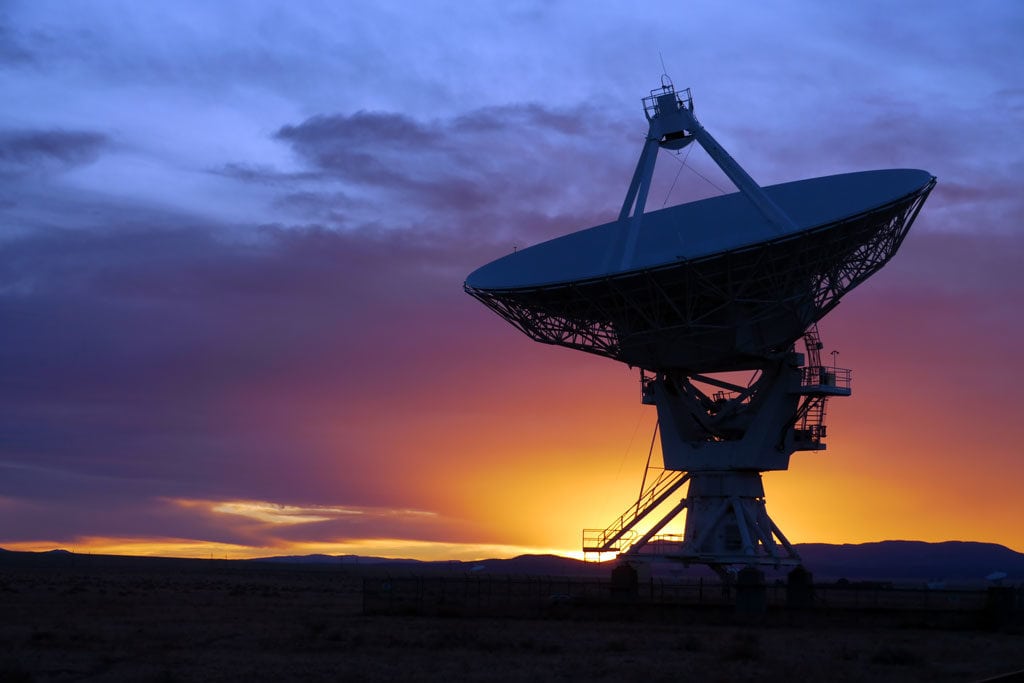This photograph, a breathtaking capture of a large radio telescope in the middle of a desert, showcases the drama of a sunset. The enormous white metal structure, resembling a giant satellite dish with a large bowl-like top, points towards the darkening sky. The intricate design features a stairwell that snakes around the structure, leading to the top, and it appears mounted on wheels for transport. Surrounding the base is a short metal fence. The telescope stands starkly against a backdrop of a sun setting behind a distant mountain range, casting a golden pinkish hue across the clouds. The sky transitions from the brilliant yellows and reds near the horizon to deep blues at the top, and the scene is reflected on the black ground. Clouds show varying shades as they fade into the night, creating a dramatic silhouette of the telescope. The entire scene is bathed in the subtle illumination of twilight, highlighting the stunning contrast and making the photograph a vivid portrayal of technology amid natural beauty.